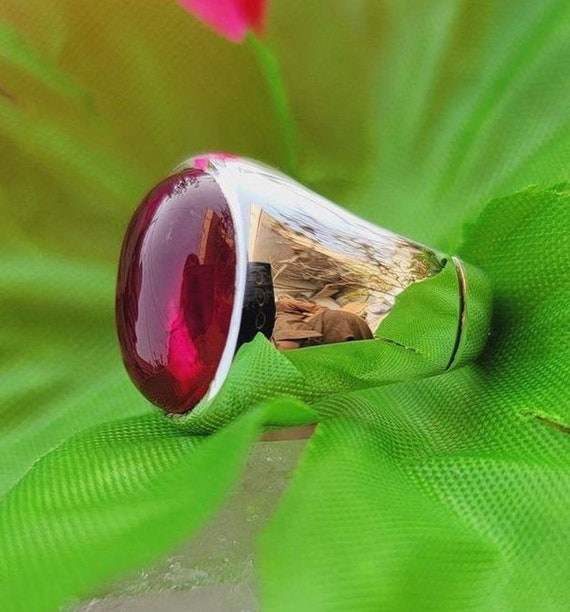The image showcases an extreme close-up photograph of a wide, golden ring sitting on its side atop a bright, green surface that appears to be a sheer, neon-green fabric or possibly an artificial leaf. The ring is partially wrapped with a green film covering the base and sits against a predominantly green background that includes a small red triangle or flower at the top. The ring features a circular red or fuchsia dome-shaped stone set into its center. Both the golden ring and the vibrant stone exhibit reflective properties, capturing and distorting images within them. The reflections within the ring and stone are somewhat unclear but seem to depict elements like a stereo system, possibly a building, people, and natural elements such as the sky and plant material. The overall scene gives the impression of a detailed, intricate piece of jewelry displayed against a vivid, spring-like backdrop.